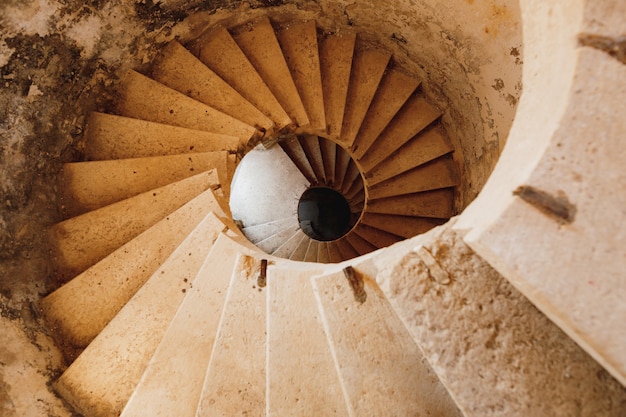This image is a detailed color photograph of a spiral stone staircase. Captured from an overhead view looking down from the top of a narrow, round tower or turret, the beige to sand-colored stone steps curve gracefully downwards, starting from the top right corner of the picture. The staircase completes around four visible levels of the spiral, although it fades into darkness beyond that point, obscuring further details. Each step shows signs of aging and wear, with imperfections, blemishes, and water stains marking their surfaces. The absence of handrails on both the inner and outer sides of the staircase adds to the sense of antiquity and abandonment. The entire scene evokes an aged, historic atmosphere, with the stone walls also bearing marks of time, featuring a range of tones from light to darker beige, giving the impression of a relic from a bygone era. There are no people, animals, or objects present in the image, emphasizing the staircase's solitude and timelessness.